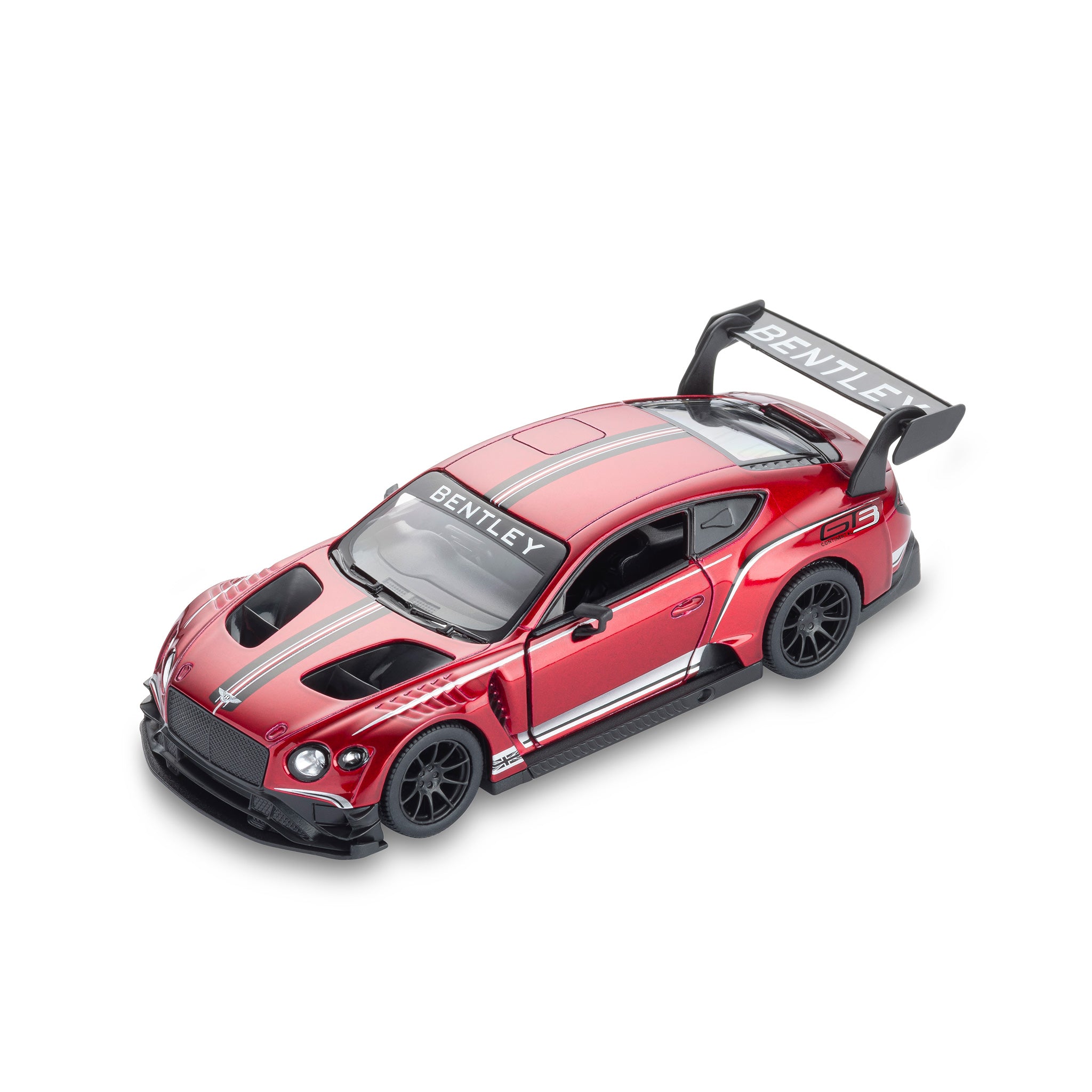This close-up photograph showcases a red, two-door model Bentley sports car set against a stark white background. The car is angled with the front engine positioned towards the bottom left corner and the rear angled towards the top right, highlighting its sleek design. The Bentley logo is prominently displayed on the front of the car. Black and white accents detail the car, including a striking black grille and black wheels with black rims.

A distinctive black spoiler is mounted over the trunk area, emblazoned with "Bentley" in white capital letters. The same "Bentley" lettering appears on a black banner across the top of the windshield. The car features a white streak along the side doors and a combination of white and black stripes running along the bottom side. There are notable design details, such as holes in the front engine portion and a black streak with a red line running down the center of the hood and roof.

The car is designed without side windows, emphasizing its sporty aesthetic. On the rear side of the vehicle, it reads "GT" in black letters and "3" in white, indicating the GT3 model. The details and decals make this model a detailed and attractive representation of a Bentley sports car.